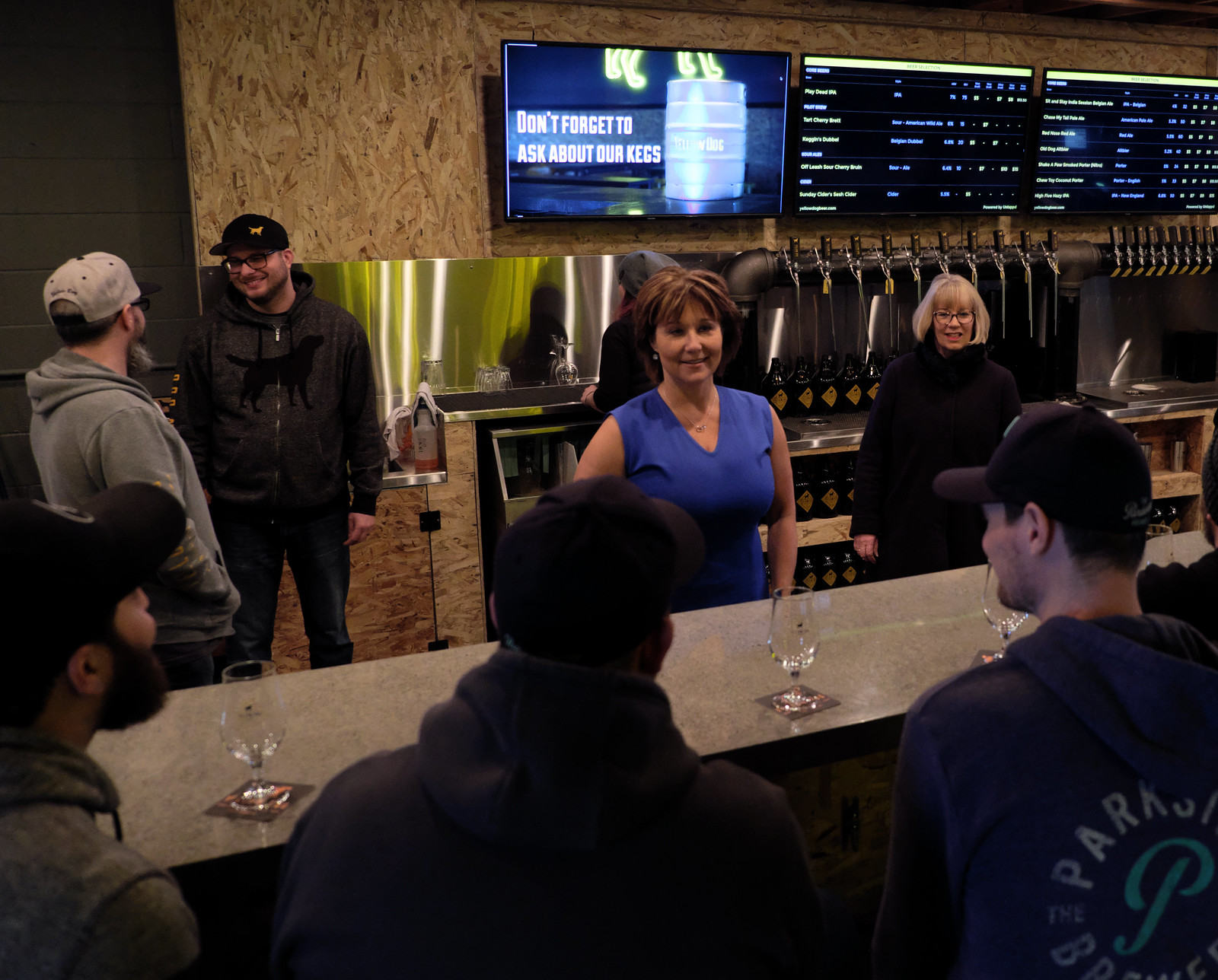This detailed photograph captures an upscale, modern indoor bar setting. Three men, casually dressed in hoodies and baseball caps, are seated at the long counter with empty wine glasses on coasters in front of them. They appear to be waiting for service, as none of them are drinking. Behind the bar stands a smiling bartender, a woman with very short reddish-brown hair, adorned with earrings, and wearing a tight, sleeveless blue blouse. She is engaged in conversation with the men. 

Next to her is another woman with short grayish-blonde hair and bangs, wearing glasses, and dressed in black. She is also smiling and looking at the men. The backdrop of the bar features a shiny, clean backsplash lined with numerous identical bottles, likely wine or growlers, and several beer taps. The back wall appears unfinished, with exposed particle board and a large roll-up gate on the far left. Overhead, there are lit screens, one of which reads, "Don't forget to ask about our kegs," emphasizing the establishment's offerings. The image captures a moment of anticipation and interaction in a sleek, contemporary bar atmosphere.